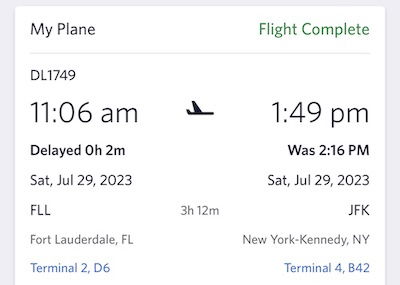The image showcases an itinerary app interface, illustrating the details of a completed flight. The app features a clean design with a white panel framed by a subtle drop shadow against a light gray or possibly light pink background, making it visually appealing yet simple.

In the upper left corner, a plane icon indicates the travel mode, accompanied by the text "Flight Complete" in green on its right, signifying the completion status of the flight. Below this header, a thin divider line separates it from the detailed flight information.

On the left side of the panel, you'll find "DL1749", which appears to be the flight number, and "11:06 AM" marked as the departure time. Beneath these details, "Saturday, July 29th, 2023" is displayed prominently, followed by "FLL" signifying Fort Lauderdale, Florida as the departure city. Terminal and gate information are provided in blue text as "Terminal 2, D6".

The right side mirrors the left's textual structuring but aligned to the right. It starts with "149 PM" indicating the arrival time, followed by "Delayed: 0 hours, 2 minutes". The initially scheduled arrival time is noted as "2:16 PM". The same date, "Saturday, July 29th, 2023", confirms the timeline. The destination is displayed with "JFK", standing for John F. Kennedy Airport, New York, with an arrival duration of "3 hours, 12 minutes". The terminal and gate at JFK are specified as "Terminal 4, B42".

Centrally placed between the left and right aligned text is a black plane icon, above the flight duration of "3 hours, 12 minutes", effectively tying the departure and arrival information together.

Overall, the clean and organized layout efficiently delivers comprehensive flight details at a glance.